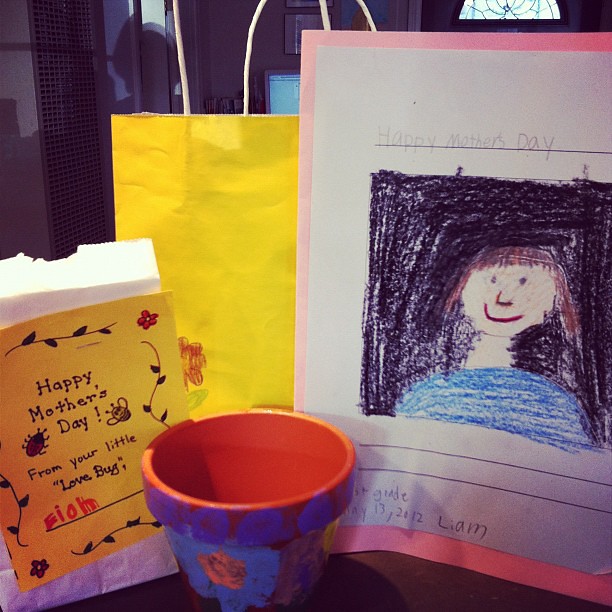This detailed indoor photo features a heartfelt display of a child’s artwork created for Mother's Day, set against a backdrop of a brown door with some shadowing. Central to the display is a white bag adorned with a yellow paper that showcases a charming drawing of a bee, a ladybug, a flower, and some vines, with the heartfelt message, "Happy Mother's Day from your little lovebug E-I-O-H," handwritten by the child. Beside this, a bright yellow bag with a crayon-drawn flower adds a burst of color.

To the right, a meticulously crafted Mother's Day picture is mounted, featuring a white sheet of paper framed by pink construction paper. The top of the white paper bears the cheerful inscription "Happy Mother's Day" in a child’s earnest handwriting. Below this, a drawing depicts a smiling mother with a longer hairstyle, dressed in a blue shirt, standing against a black background. The drawing is identified with the child’s name and the date at the bottom. To the left of the display, a painted flower pot holds a blue flower, showing the child’s artistic effort with strokes of various blues and browns. This delightful array of crafts and drawings exudes warmth and the genuine affection of a child’s love for their mother.